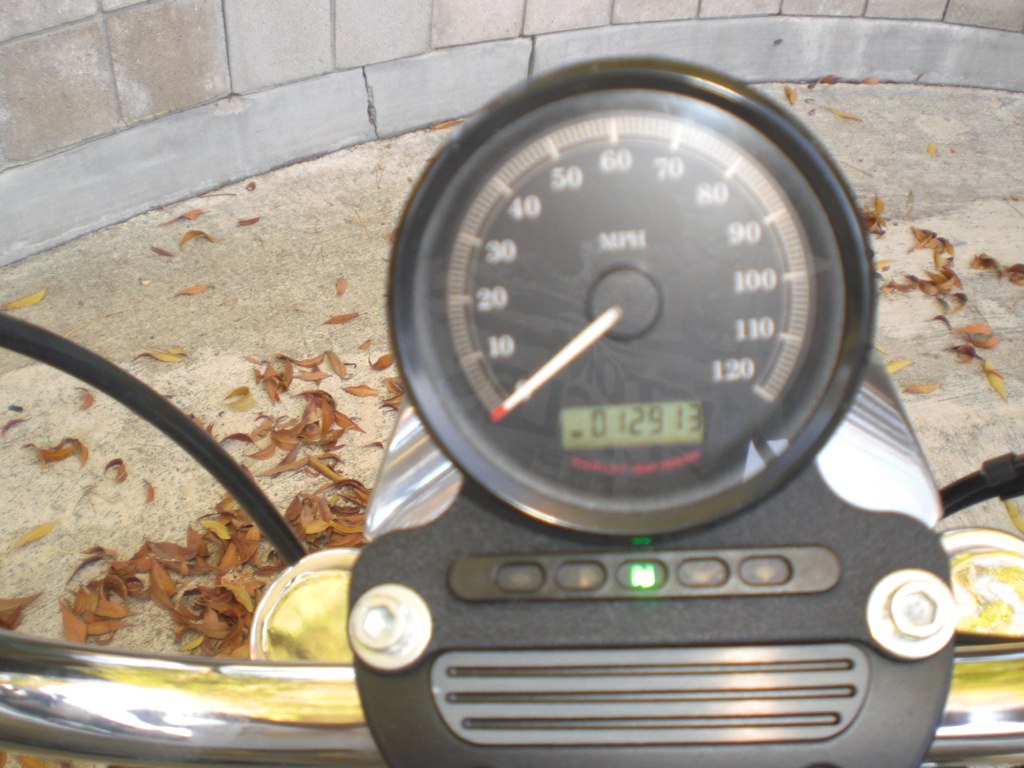The photograph captures a close-up view of a speedometer and odometer mounted on the handlebars of an unspecified vehicle, possibly a bike or a snowmobile. The speedometer displays the speed in miles per hour, while the odometer below it records the total miles traveled. The focus is on the large dial, obscuring the front of the vehicle and leaving its true nature unidentified. The handlebars are attached to a console featuring two prominent bolts and several indicator lights. Chrome handlebars extend outwards on both sides, with visible cabling, potentially for the brake and clutch systems. The background includes a cinder block wall, light-colored sand, and scattered fallen leaves, adding detail to the setting.